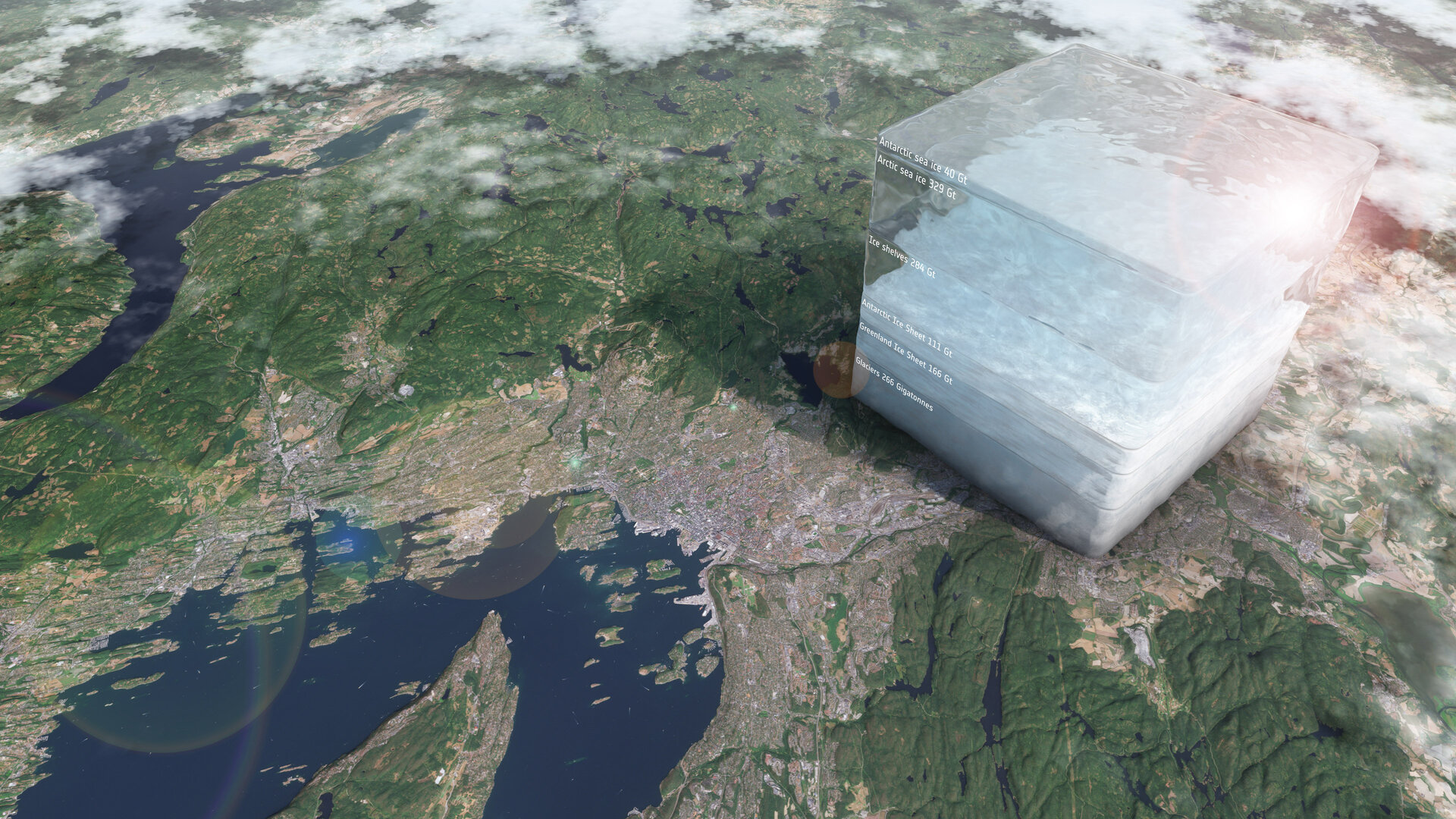The image is a large, color 3D rendering, depicting an informational graph in the form of a detailed, miniature geographical map viewed from space. The map showcases a large, green landmass transitioning to brown along the coast and surrounding a large, blue bay of water. Small islands dot the water, and scattered white clouds partially obscure the view, with bright sunlight illuminating the scene from the right. 

Prominently positioned in the top right, a series of massive, layered cubes—each representing different forms of ice—are stacked, their sheer size dwarfing the city below. The white box-like structure, resembling glass or plastic, illustrates the volume of ice visually through its various labeled layers: Antarctic Sea Ice (40 GT), Arctic Sea Ice (329 GT), Ice Shelves (284 GT), Antarctic Ice Sheet (111 GT), Greenland Ice Sheet (166 GT), and Glaciers (266 GT). The render gives a clear, textured impression of the scale and mass of these ice forms, juxtaposed against the map’s terrestrial and aquatic features to convey the immense quantities of ice in a strikingly visual manner.